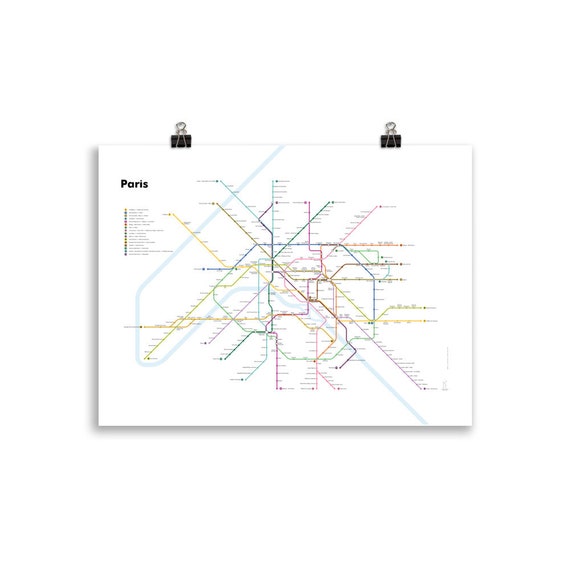This detailed image features a color illustration in a landscape orientation, showcasing a detailed subway map of Paris, France. The map occupies the central area, bordered by a gray frame and set against a white background. The map itself is rich with intersecting lines that represent various routes of the Paris public transportation system. These lines come in vivid colors: pink, purple, green, yellow, blue, and black, each leading to different locations and points of interest. At the top left corner of the map, the word "Paris" is prominently displayed in bold black text. Beneath the title is a column of text labels, which serve as a color key for the map, although the text is too small to be readable.

The top edge of the map is secured with two black binder clips, one on the left and one on the right, holding it firmly in place. The map is designed with a slightly three-dimensional effect, having a drop shadow on the left side and across the bottom, giving it a floating appearance. Overall, this illustration serves as an informational chart, meticulously detailing the subway routes across Paris with color-coded lines and textual annotations.